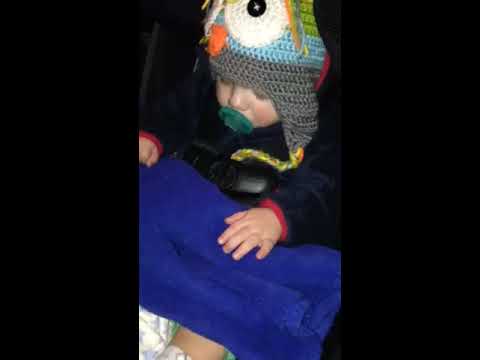This photograph is a small, heavily pixelated close-up of a young light-skinned child, likely a baby transitioning to toddlerhood, sitting in a car seat. The image captures the child from head to toe, with black bars on the sides indicating a cropped, portrait orientation. The child is wearing a dark blue fleece jacket with red trim on the cuffs and hood, and his or her hands are outstretched, resting on a deep blue, fuzzy fleece blanket that partially covers their legs, one of which peeks out from the bottom left corner of the image.

The child has a large green pacifier in their mouth and is wearing a colorful knitted cap with ear flaps that tie under the chin. The hat features distinctive owl-like details: two large white eyes with black button pupils and an orange beak, with the lower half of the hat being gray, the center blue, and the top green. The child appears calm, possibly sleeping or focused on something beneath the blue blanket. The scene is further framed by the black plastic locking mechanism of the car seat, clearly securing the child in place.